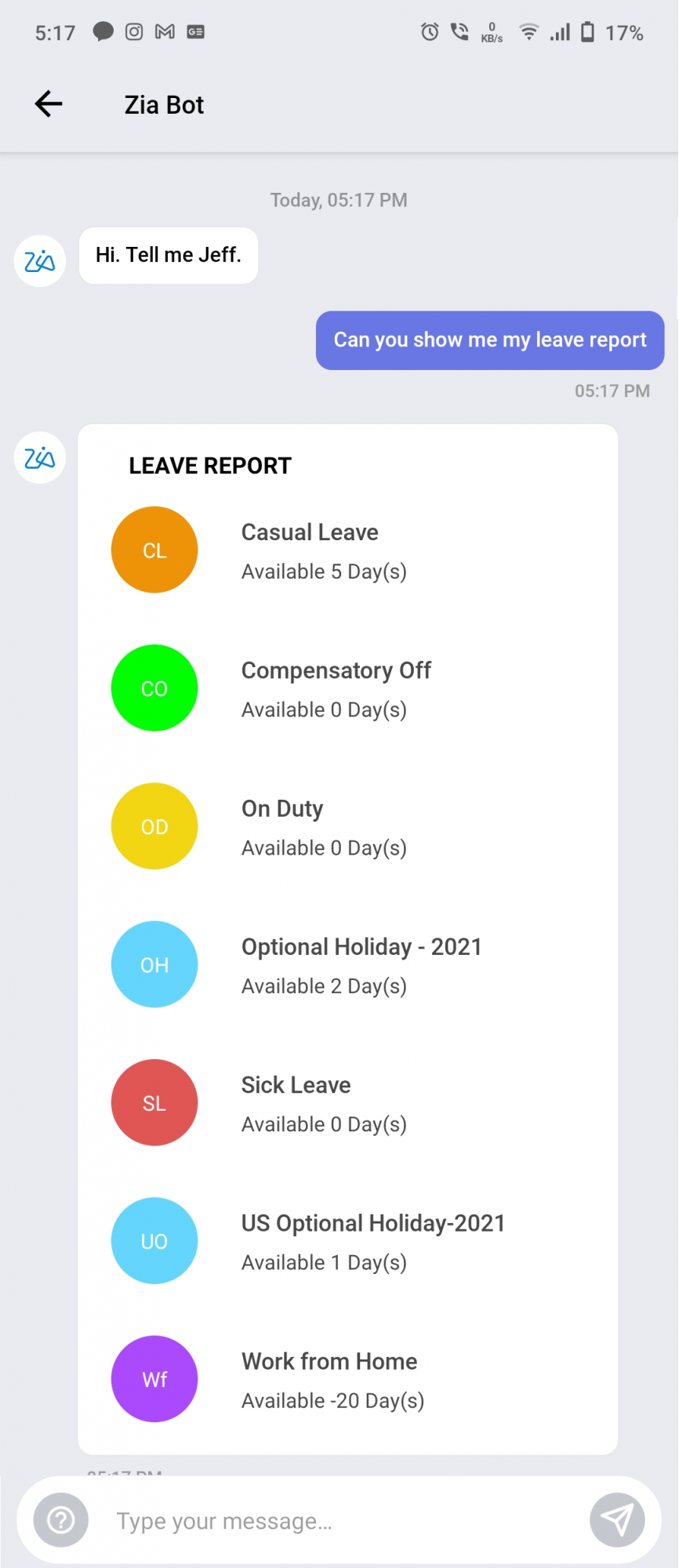The image is a screenshot of a smartphone interface with a gray background. At the top part of the screen, in a darker shade of gray, the time is displayed as 5:17 PM. Below the time, a notification bar contains various app icons: the Instagram logo (a camera lens), the Gmail logo (an envelope with an "N"), and another unidentified app with a "G" inside a rectangle. Additionally, there is a log file icon showing "0 KBS" with the phone battery level at 17%.

On the left side, underneath this row of icons, a black arrow points to the left, with the text "ZiaBot" next to it in black. Following this, a thin gray line separates the date and time, displayed as "Today, 05:17 PM". 

Further down, there is a conversation interface featuring a white circle logo of ZiaBot, characterized by a blue "Z" with a squiggly line within it. Adjacent to the logo is a white message bubble with black text saying "Hi, tell me Jeff." On the right, a purple message bubble contains white text reading "Can you show me my leave report at 05:17 PM". 

This is followed by ZiaBot's response in a white message bubble with black text, labeled "Leave Report": 
- Casual Leave: Available 5 days
- Compensated Off: Available 0 days
- On Duty: Available 0 days
- Optional Holiday 2021: Available 2 days
- Sick Leave: Available 0 days
- U.S. Optional Holiday 2021: Available 1 day off
- Work from Home: Available 20 days off